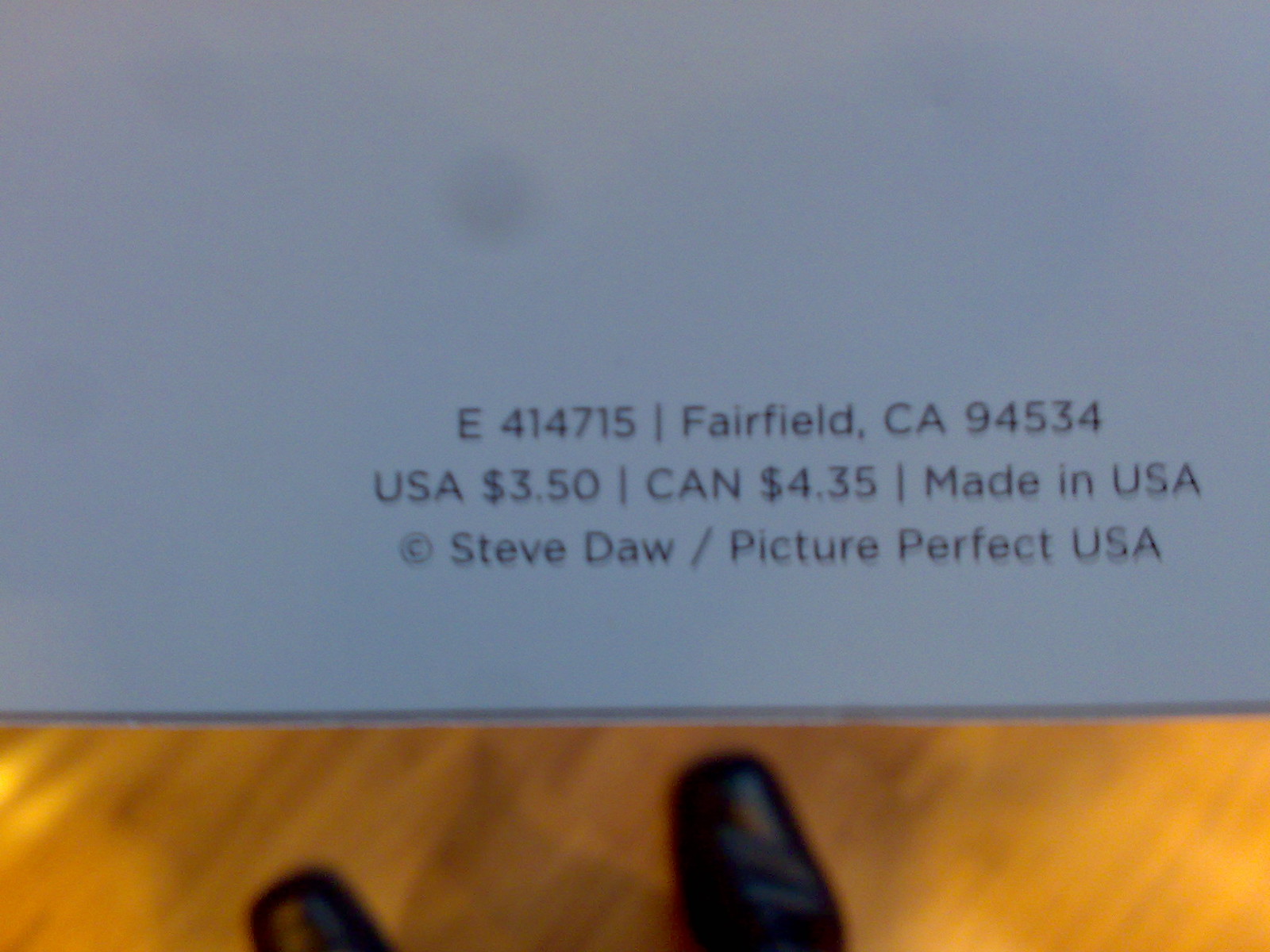The photograph captures a card with black text on a grey background, which reads "E414715, Fairfield, California 94534, USA $3.50, CAN $4.35, Made in the USA, © Steve Dahl, Slash Picture Perfect USA." The image includes a hardwood floor and the tips of someone's square-toed black leather shoes, slightly visible from the bottom edge. The text appears somewhat blurry, potentially due to the lighting conditions when the photo was taken.